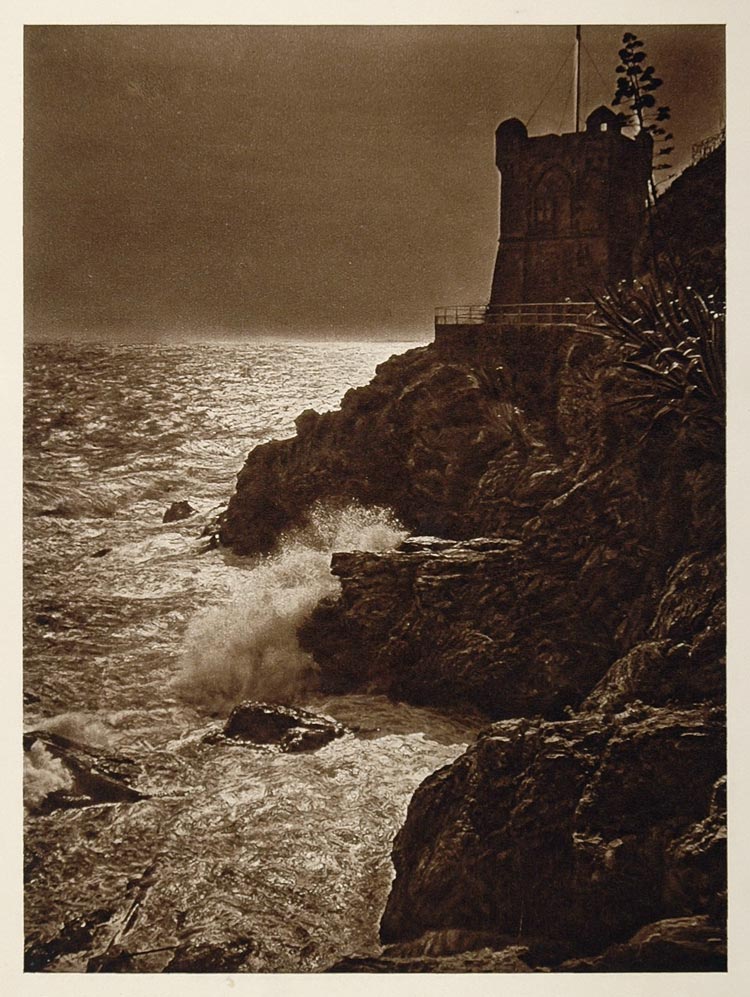This image depicts a vintage sepia-toned photograph bordered in white, possibly from the early 1900s. The scene captures a rugged coastal landscape with a steep, rocky shoreline. On the left, powerful waves crash against the rocks, creating a striking contrast with the calm, clear sky occupying the top third of the image. Dominating the upper right portion of the scene is a two-story stone structure resembling a castle tower or lighthouse. This tower, perched precariously on the edge of the cliff, features a metal pole atop and an outdoor balcony with a modern railing. Surrounding the tower are splashes of greenery, including a tree and various plants, adding a touch of life to the stark, dramatic scenery.